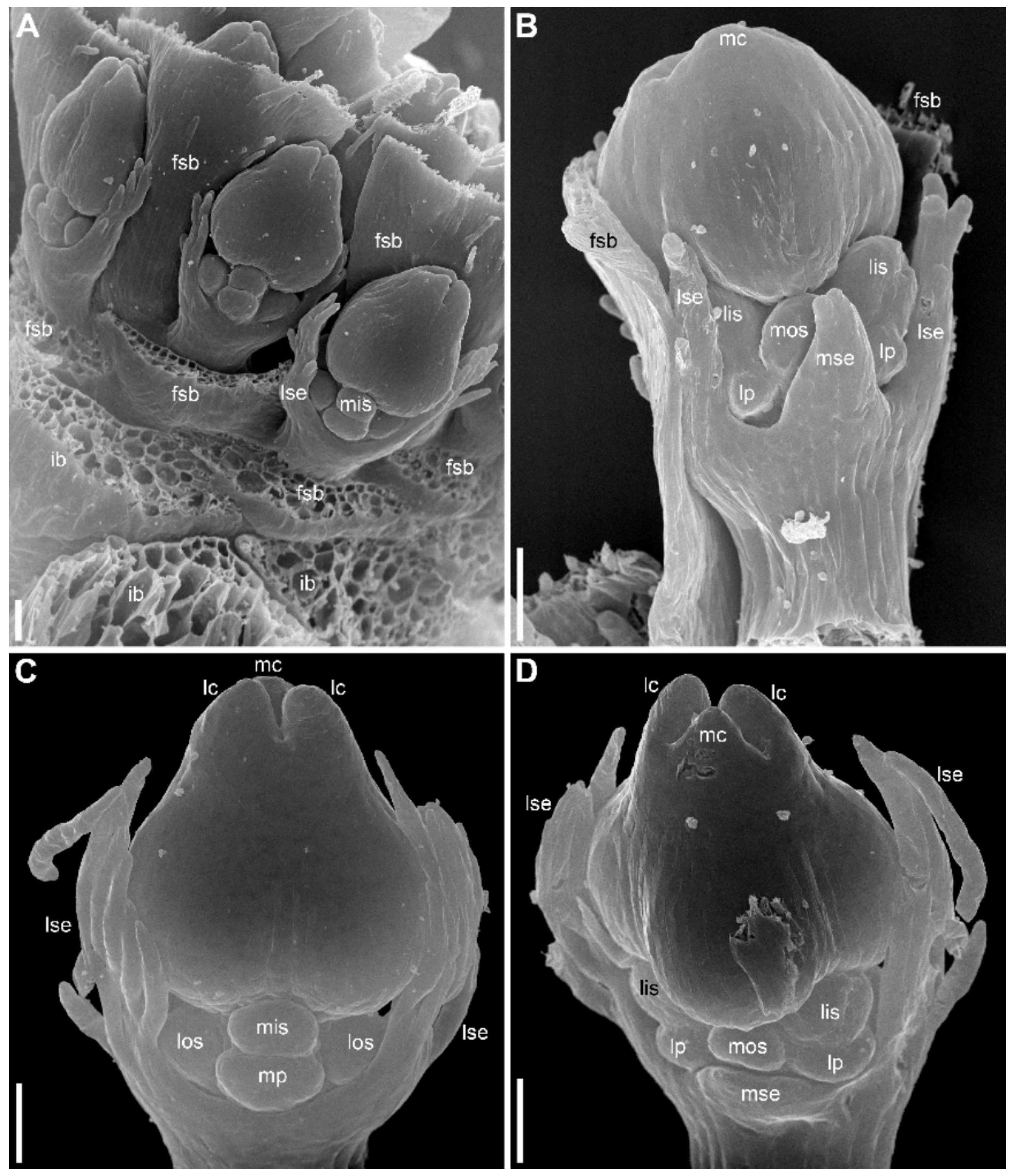The image is a vertical rectangular composite of four smaller vertical rectangles, each delineated by a thin white line. Arranged in a grid pattern, these sub-images are labeled with white capital letters A, B, C, and D, positioned in the upper left corner of each section. All four images resemble x-ray or SEM scans with numerous three-letter labels such as FSB, MIS, IB, and LSE scattered across various structural features. 

Image A, in the upper left, presents a zoomed-in view with gray, petal-like structures transitioning into a spongy texture below, displaying visible pores. Image B, in the upper right, has a solid black background, featuring a different angle of the same structure seen in A, perhaps likened to a fragmented bone or intricate floral petal, also marked with labels such as FSB, LSC, LIS, and MOS.

Images C and D, located at the bottom left and right respectively, maintain the black background and showcase alternative perspectives of the mysterious object, which could be hypothesized as bone or organic material due to its textured appearance and cavity-like formations. These images, including labels like MP, LOS, and LSE, progressively darken in tone, enhancing the depth and complexity of the featured structures.